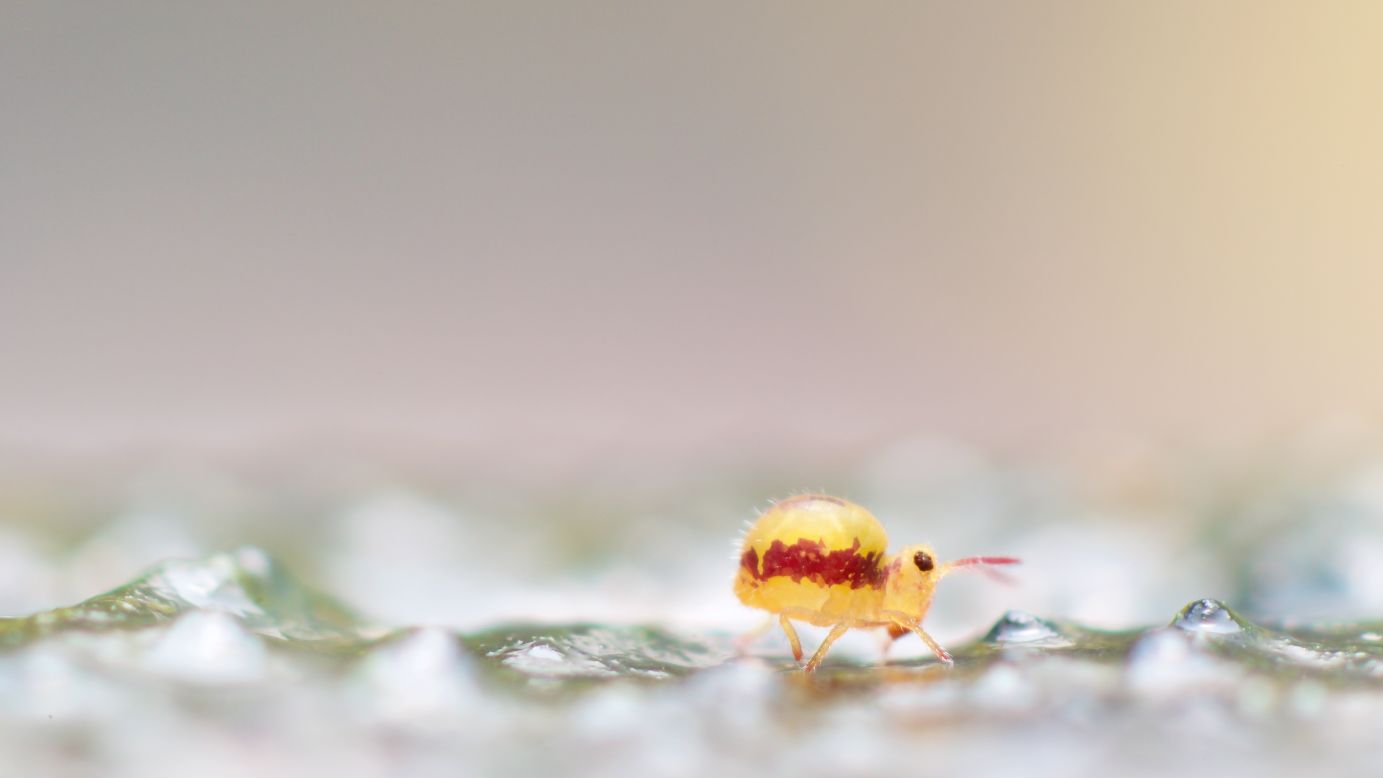The image depicts a highly magnified close-up of a small insect, vividly detailed against a blurred background. The insect, which appears to be a beetle or ladybug, is bright yellow with a distinct horizontal red stripe encircling its body. Its prominent black eyes and reddish antennae add to its striking features. The insect is positioned straight-on, standing on top of water which forms bubbles and splashes around it. The background colors blend into muted tones of pink, blue, and green, creating an ethereal backdrop that contrasts with the sharp clarity and brilliant colors of the insect in the foreground. The exact setting is ambiguous, but the insect's ability to walk on water suggests a natural, outdoor environment, possibly a puddle or a small body of water.